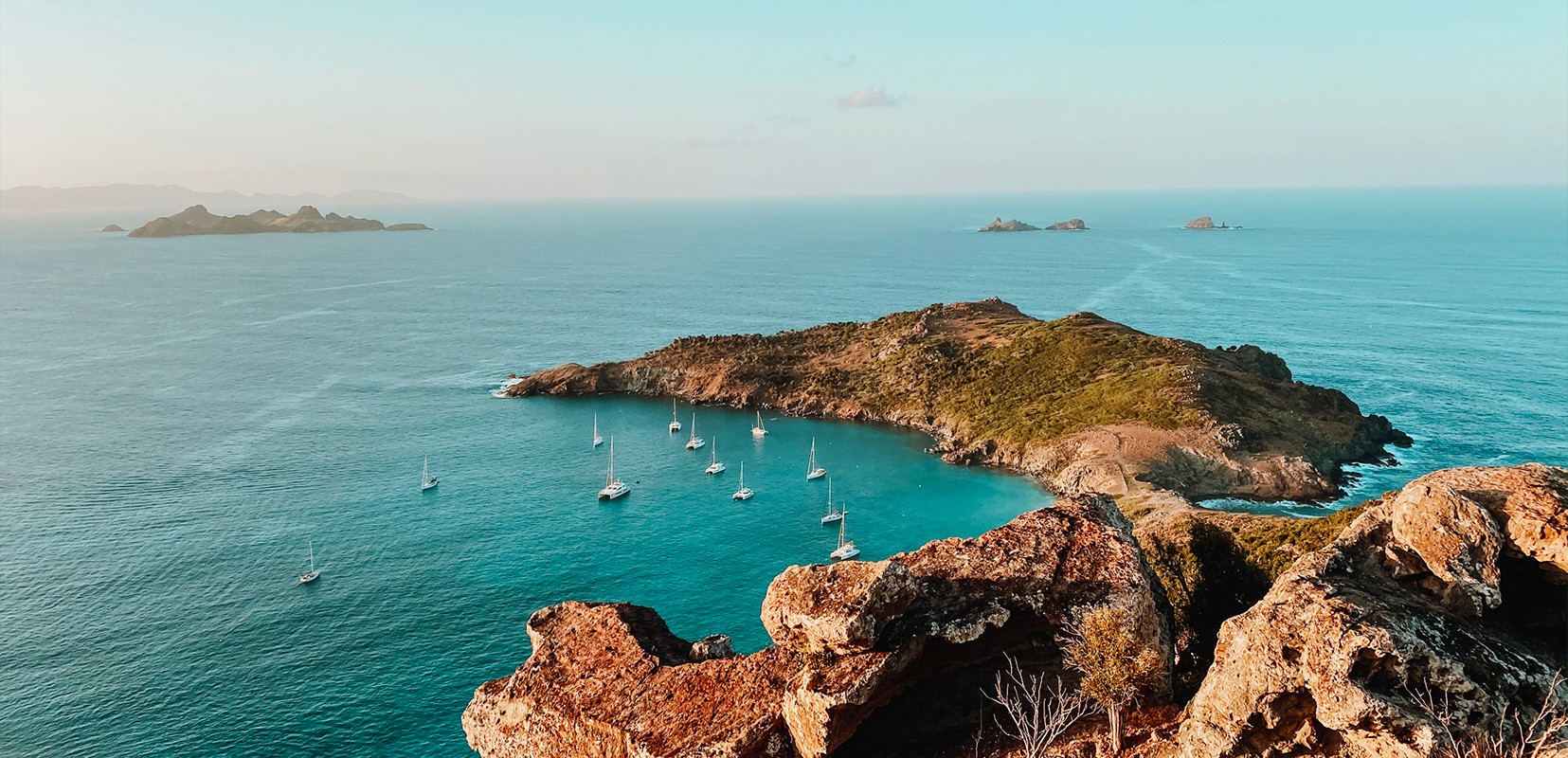This image captures a stunning aerial view of a vibrant blue ocean, dotted with four picturesque islands. Taken from a high vantage point on a larger island, the photo's angle slightly inclines downward, offering a comprehensive perspective. In the background, the horizon blends the sky with the sea, highlighting the expanse of the landscape. To the right, about a third from the top of the frame, an elongated island stretches from left to right, flanked by two smaller, rocky protrusions. 

Closer to the foreground, a modest-sized island covered in grass and a few trees sits, with its serene shores attracting a fleet of approximately twelve small boats, likely fishing vessels. These boats are positioned near the island, adding a sense of scale and activity to the tranquil scene. The bottom portion of the image features jagged rocks that sweep from the right to about two-thirds across the photo, leading the viewer’s eyes back into the expansive ocean. The absence of human structures or people on these islands preserves the untouched and natural beauty of this captivating seascape.